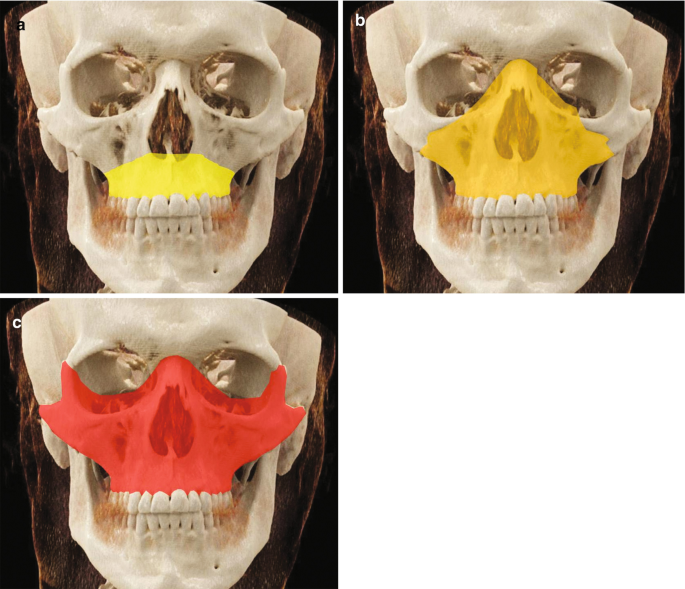The image is a collage divided into four quadrants, three of which contain x-ray images of a human skull, while the fourth, located at the bottom right, is empty. Each x-ray image is of the same skull, focusing from the forehead down to the jaw, and is labeled consecutively: 'A' for the top left, 'B' for the top right, and 'C' for the bottom left. 

Image A features a yellow-highlighted area just above the upper teeth, where the upper lip would be. In image B, the yellow extends to cover the upper lip, nose, and the area below the eyes and both cheeks. Image C shows a red-highlighted region that spans from the nose to the ears, covering the upper lip, cheeks, and the lower parts of the eyes. The skulls in the images are white, typical of x-ray visuals, with the highlighted areas possibly indicating regions of interest such as hot spots or areas of infection.